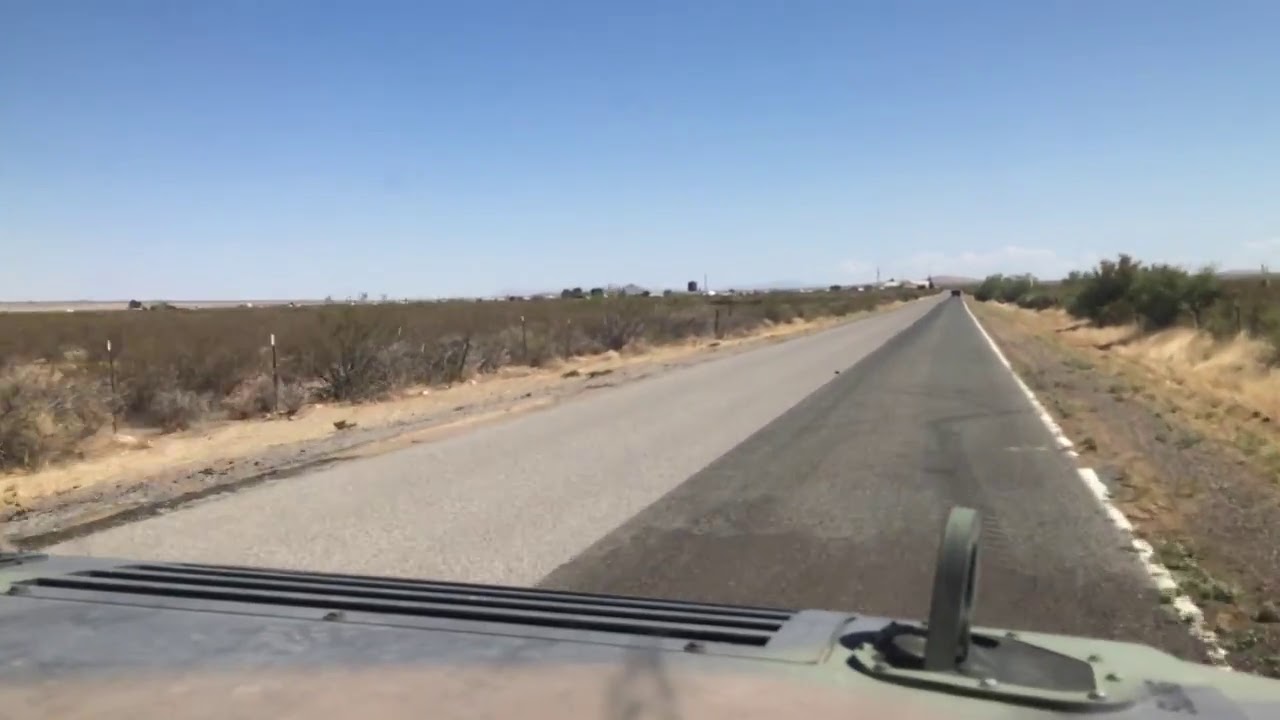The image captures GoPro footage from the top of a car, showcasing a long, paved road that stretches into the horizon. The roof of the car, partially visible and metallic, hints at the viewer's perspective from atop the vehicle. The road is distinctive, divided into two lanes: a darker, blackish section on the right and a lighter, grayish section on the left, separated by a central white line. On both sides of the road, the landscape is flat and arid, populated with sparse bushes and patches of dead grass, indicating a dry climate. The left side appears more sunbaked with a thin, almost invisible fence marking the boundary, while the right side shows slightly more greenery amidst the dry terrain. In the distance, there's a solitary car seemingly miles ahead, underscoring the vast openness of the scene. The sky is a clear, deep blue with occasional light clouds. On the horizon, a cluster of small buildings hints at a potential town, rest stop, or farm, breaking the monotony of the flat landscape.